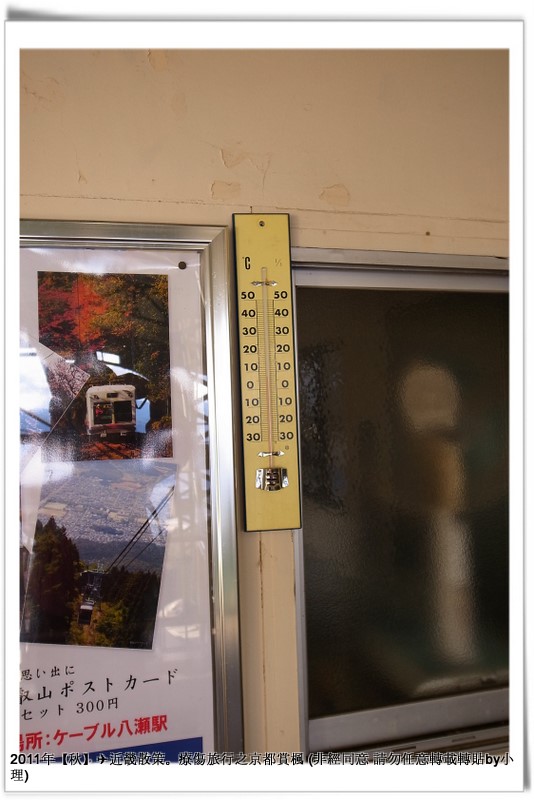The image captures an outdoor thermometer mounted on a weathered, beige-painted, wooden wall. The paint on the wall shows signs of aging, characterized by peeling in several areas, revealing the wooden texture beneath. The scene is bathed in abundant natural sunlight, which casts reflections that enhance the outdoor setting. 

To the right of the thermometer, there's a frosted glass window reflecting sunlight, adding to the ambiance. On the left side, a plastic-covered advertisement with some photos also reflects light, contributing to the bright, well-lit scene.

The thermometer, narrow and rectangular, shows temperature in Celsius with markings starting at 50 degrees and moving down in increments of 10 degrees to -10 degrees, then upwards again. Unfortunately, the angle of the photo does not allow for a clear reading of the current temperature.

Below the thermometer, the year "2011" is prominently displayed, accompanied by numerous Chinese characters in black, suggesting that this thermometer was likely made or installed in that year. The presence of these characters hints at an East Asian context for the scene.